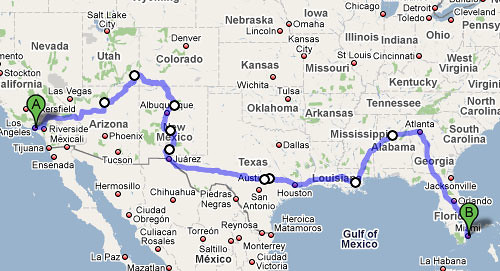This image depicts a detailed map of the United States with a highlighted driving route. The journey commences at point A in Los Angeles, California and proceeds eastward. The first stop on this extensive trip is in Arizona, followed by a stop in Utah. The route then heads southward with stops in Albuquerque, New Mexico, and Juarez. Continuing east, the route includes stops in Austin, Texas, and then further east into Louisiana. The journey progresses through Alabama with another stop, moves on to Atlanta, Georgia, and subsequently reaches Florida with stops in both Jacksonville and Orlando. The final destination of this comprehensive road trip is Miami, Florida. The map provides a broad view of the United States, emphasizing the transition from the southwestern states to the southeastern regions, showcasing a thorough cross-country drive.